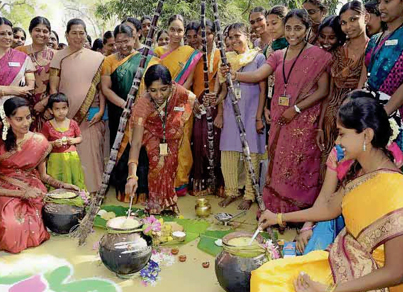In this vivid daytime scene set outdoors, a large group of around thirty people, predominantly women, are gathered around a cooking area. They are all adorned in vibrant, traditional Indian attire featuring colorful saris in shades of pink, red, yellow, light purple, and light green. The image, a color photograph with a landscape orientation, captures the cultural essence of the moment, portraying the participants engaged in a communal cooking activity. In the center of the photograph, a woman bends over to stir a pot on the ground using a stick, while another woman on the right side, seated and in profile, also stirs a pot. These pots, which sit on a mat with a floral design, are arranged beneath a sturdy tripod made of dark-colored bamboo sticks. The ground is adorned with various scattered objects and is painted in lively hues of green and pink, enhancing the cheerful ambiance. Among the attendees, some women wear name tags attached either to black lanyards or directly to their clothing. In the background, a line of trees frames the energetic scene, completing this colorful and culturally rich tableau.